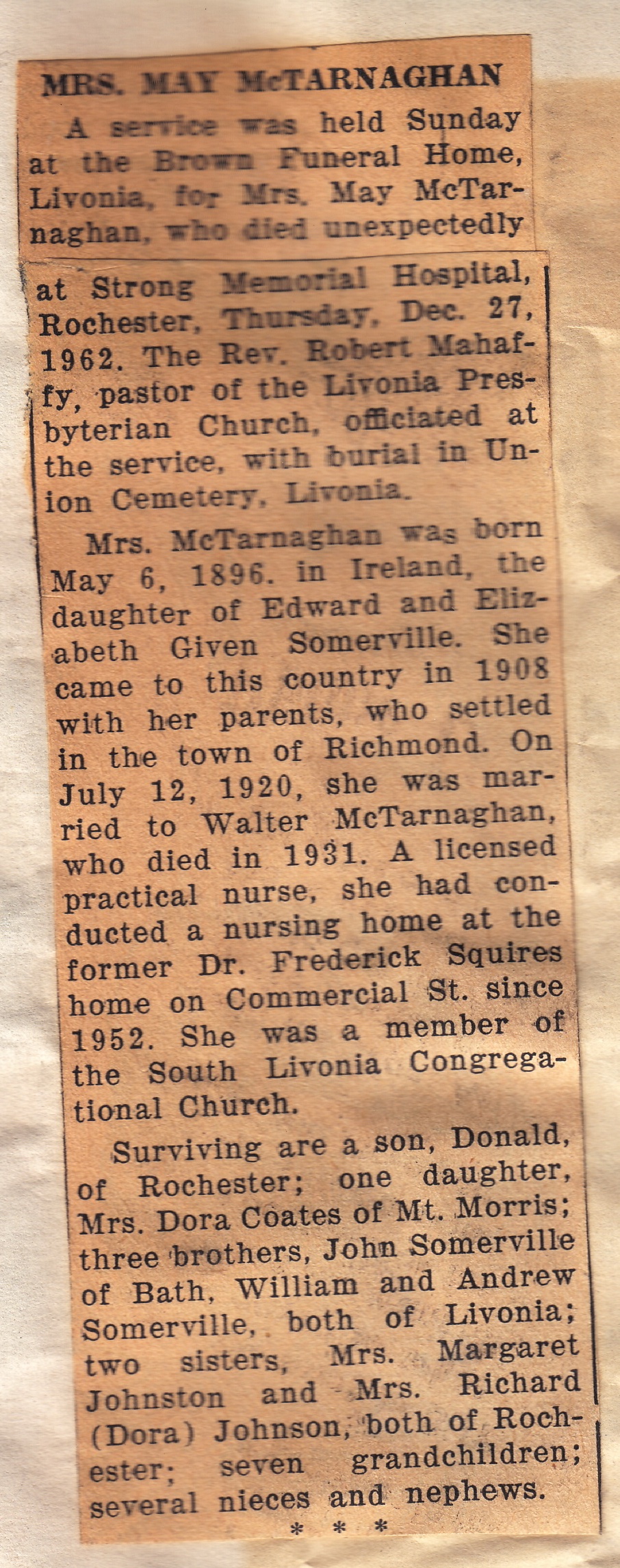The image depicts a tall, narrow newspaper clipping, browned with age, containing the obituary of Mrs. May McTarnaghan. The text is set against a whitish paper background. At the top, in bold black print, it reads "Mrs. May McTarnaghan." The obituary announces that a service was held Sunday at the Brown Funeral Home in Livonia for Mrs. McTarnaghan, who passed away unexpectedly on Thursday, December 27, 1962, at Strong Memorial Hospital in Rochester. The officiant of the service was Reverend Robert Mahaffey, pastor of the Livonia Presbyterian Church, and the burial took place at Union Cemetery in Livonia.

Mrs. McTarnaghan was born on May 6, 1896, in Ireland, the daughter of Edward and Elizabeth Given Somerville. She immigrated to the United States with her parents in 1908, where they settled in the town of Richmond. On July 12, 1920, she married Walter McTarnaghan, who predeceased her in 1931. A licensed practical nurse, Mrs. McTarnaghan operated a nursing home at the former residence of Dr. Frederick Squire on Commercial Street since 1952. She was a member of the South Livonia Congregational Church.

She is survived by her son, Donald, of Rochester; her daughter, Mrs. Dora Coates, of Mount Morris; three brothers, John Somerville of Bath, William Somerville, and Andrew Somerville, both of Livonia; two sisters, Mrs. Margaret Johnston and Mrs. Richard (Dora) Johnson, both of Rochester; seven grandchildren; and several nieces and nephews.